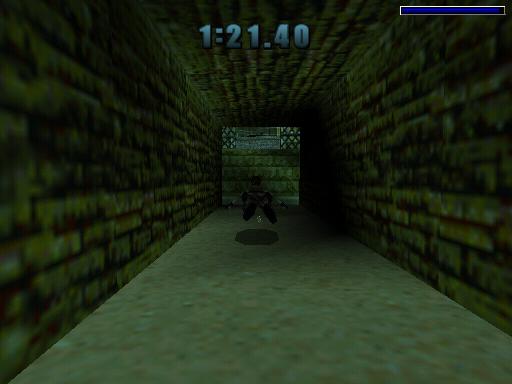This is a small screenshot from a video game with graphics reminiscent of the Nintendo 64 era. The image depicts a first-person point of view inside a tunnel constructed from brown stone, with a dirt floor. Positioned in the center of the tunnel, there's a levitating robot resembling the upper torso of Robocop, noticeably armless and casting a circular shadow below it. In the distance, the exit of the tunnel is visible, illuminated by daylight. The top of the screen displays "1:21.40" in blue font, accompanied by a small blue bar situated in the upper right corner.